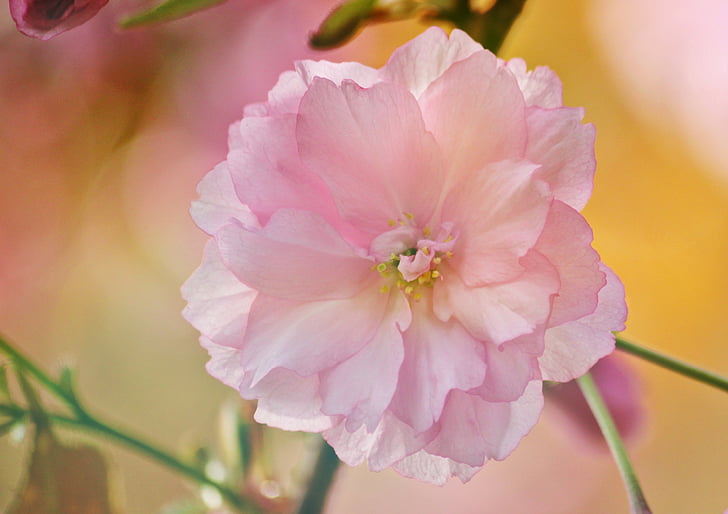This image, captured by a nature photographer, showcases a striking close-up of a delicate flower. The bloom predominantly features very light pink petals, closely packed together and slightly jagged at the edges, giving it a soft and almost velvety appearance. In the center of the flower, tiny yellow pearl-like buds, or pollen sacs, are clustered together, contrasted by hints of green. The main flower, which is the focal point, fills most of the image, with its green stem partially visible and seeming to branch off at the top, possibly supporting other blossoms.

The background is artistically blurred, cloaking the surroundings in a soft, almost dreamy overlay of yellow and pink hues. Among the blur, you can discern green stems and perhaps additional flowers of pink and red shades. The sunlight reflecting on the petals and stems indicates that the picture was taken on a sunny day, enhancing the flower's vibrant colors and the overall warm ambiance of the scene.